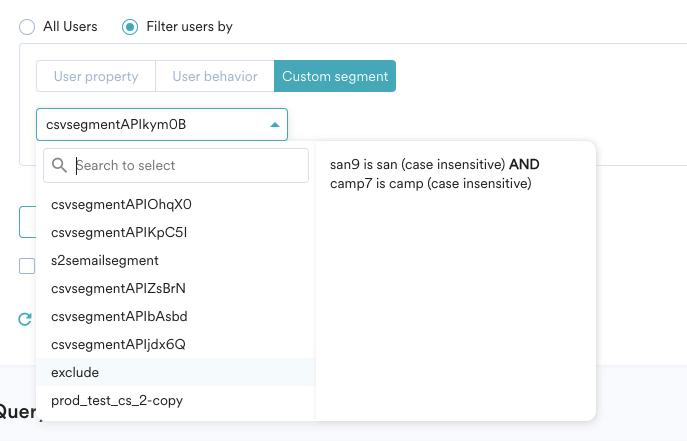This image depicts a computer search interface, likely tailored for advanced user queries or data retrieval tasks. At the top, users are given filtering options: 'All Users' or 'Filter Users By'. In this case, the user has selected 'Filter Users By', with additional refinement through the 'Custom Segment' option, indicated by the third box on the right, highlighted in green. Alternative filtering choices include 'Filter Users by User Property' and 'Filter Users by User Behavior', which appear as adjacent options.

Below the search bar, a series of search results are displayed, each consisting of long alphanumeric strings. There are approximately eight to ten such entries listed vertically on the left-hand side of the interface. Representative strings include "CVS segment", followed by sequences like "APIOHQX0", showcasing typical expressions users might employ.

On the right-hand side, there are two specific entries: "san 9" (with 'san' denoted in a case-insensitive manner) and "camp 7" (with 'camp' indicated as case-sensitive). The exact purpose of these strings is unclear; however, the interface appears designed to aid users in locating specific files or data strings within their directory or database.

Overall, this search page serves as a specialized tool for users requiring precise retrieval of complex alphanumeric data strings, possibly for organizational or computational tasks.